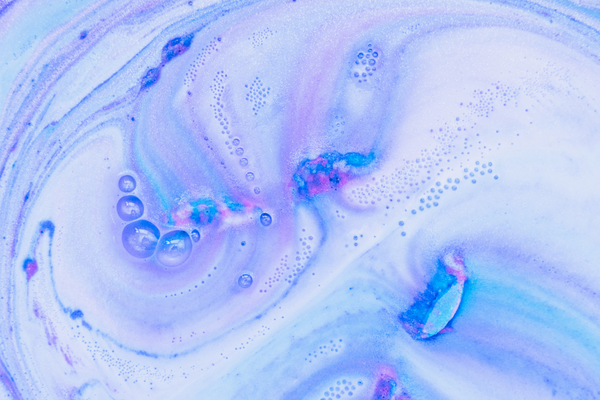The image depicts a captivating interplay of colors and textures, resembling a thick, milky liquid with a bright white base accented by blue and purple hues. Bubbles of various sizes float on the surface, adding to the frothy and viscous appearance. Swirls and thin lines of blue and purple dance across the image, creating a dynamic, almost soapy texture. The background is a light bluish tint, adding to the watery feel of the scene. In the bottom right, a large ring suggests the presence of a significant drop, while smaller yellow ring-like circles appear towards the middle left. In the center left, four bubbles spiral upwards from largest to smallest, contrasting with a prominent large half-bubble in the center right. This half-bubble magnifies the blue hues, with the top part showcasing a mesmerizing purple-pink swirl. Throughout the image, small bubbles are scattered, especially in the right middle top area, enhancing the overall impression of a soapy, bubbly, liquid scene.